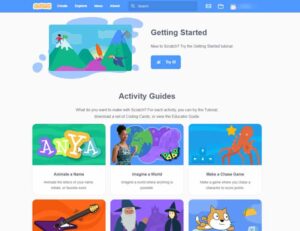This image appears to showcase a kid's website, albeit somewhat blurry and small, making it difficult to identify specific texts or finer details. In the upper left corner, there's a blue navigation bar featuring an array of options written in white text, though the words are indistinct. 

Positioned towards the top middle of the site is a visual graphic depicting mountainous terrain with a climber holding a flag and an accompanying bird in flight. The words "Get Started" are prominently displayed within this section. 

Beneath this, a section titled "Activity Guides" is visible, though some of the accompanying text is illegible. Below this section are two rows of image boxes: the first row contains three images, and the second row also has three images, though the bottom row is partially cut off, obscuring some details. 

The described images include:

1. A green background with dark and light green squiggly stripes. Superimposed are the letters "A" (white with a purple border), "N" (white with a green border), "Y" (white with a yellow border), and another "A" (white with a blue border).
2. To the right, an image features a woman standing in front of a purplish background merging into an Earth icon, accompanied by a butterfly.
3. The final image in the top row has a blue background showcasing an orange octopus paired with a yellow star.

The bottom three images are unspecified due to being cut off, rendering them partially visible.